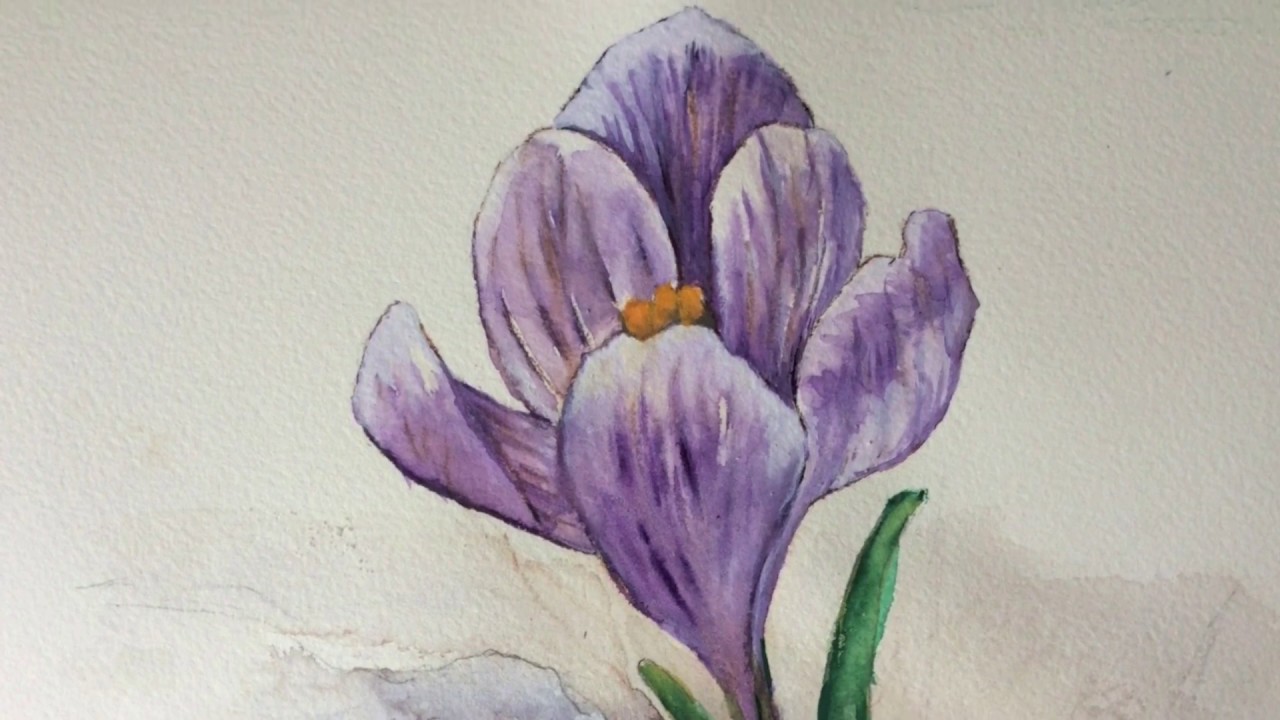A delicate sketch of a single, beautiful purple flower, centered on a cream-textured, canvas-like background with subtle brown shading at the base. The flower features six petals, primarily light lavender with hints of dark purple and white. The petals are arranged with three at the bottom, two slightly elevated above them, and one at the very top, appearing to gently close towards the center. The lower petals are slightly open, while the upper petals hug closely together. The core of the flower displays a cluster of small, yellow seed-like elements, representing pollen. Two green leaves are visible; the right leaf extends longer than the shorter left one, adding a touch of natural asymmetry to the composition. The overall effect is a harmonious blend of soft purples and greens, with a beautiful yellow accent at the heart of the flower.